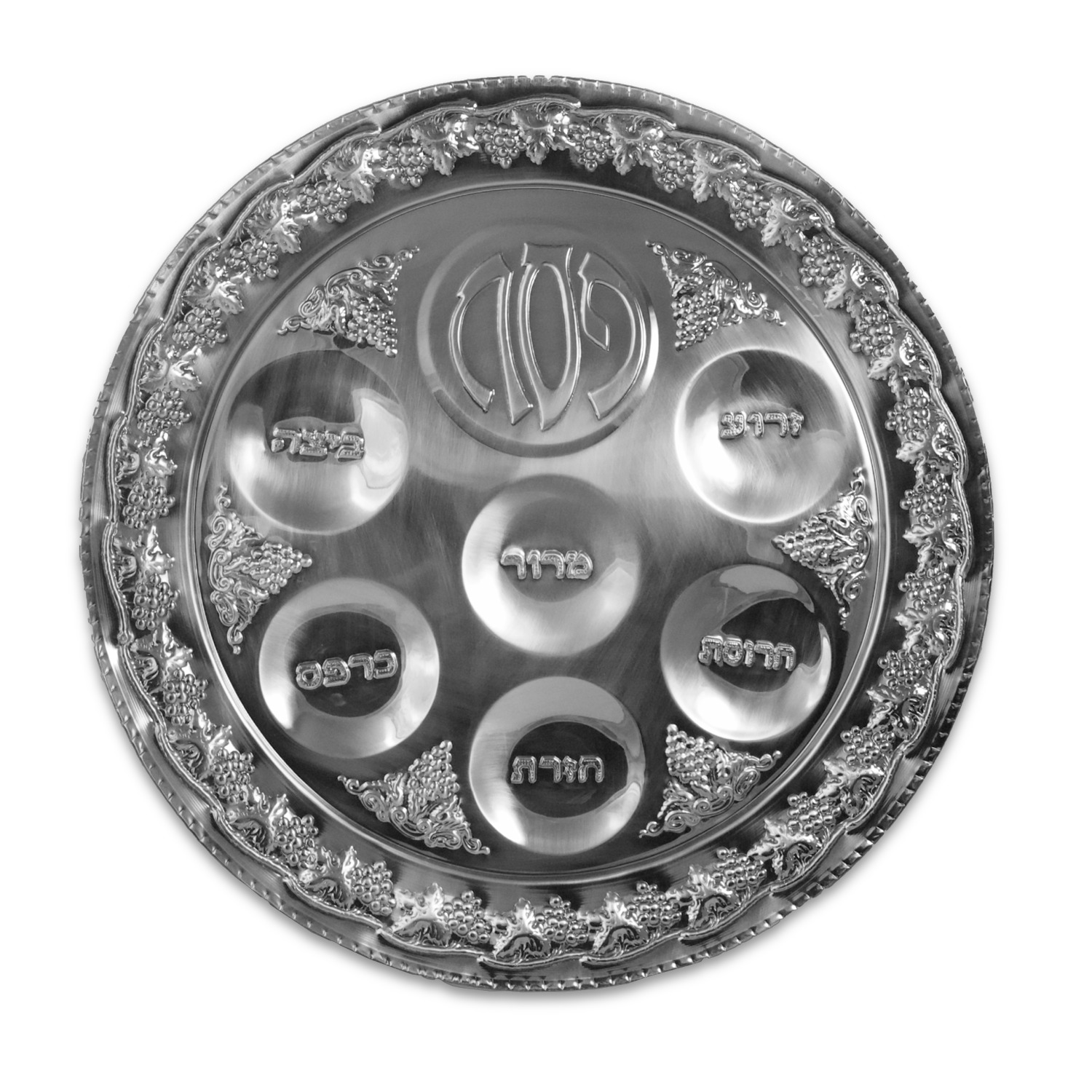This image features an ornate silver platter, potentially made from real silver or an alloy, set against a white background. The border showcases a detailed vine-like pattern of embossed grape clusters and leaves, giving it a three-dimensional effect all around the circumference. In the central area of the platter, there are seven shallow, concave discs. Six of these discs are uniform, each adorned with Hebrew script. The seventh disc, located at the top, stands out slightly, featuring raised numbers or symbols that appear to be A09 or 109 accompanied by a couple of grapes. In between each disc, decorative clusters add to the overall intricate design. The purpose of this platter remains unclear, but the presence of Hebrew lettering suggests it might have either religious or cultural significance. The image provides no additional context such as date, location, or size, and there are no labels or identifying information visible.